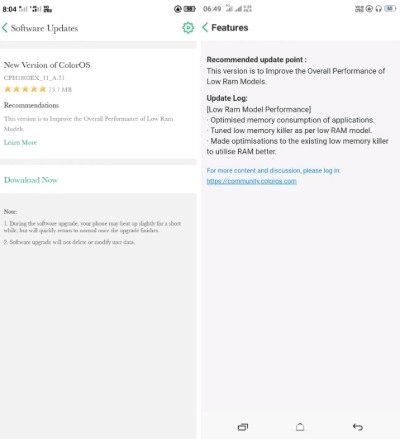This composite image consists of two smartphone screenshots placed side by side, both set against a predominantly white background.

**Left Screenshot:**

- **Headline:** "Software Updates" in bold text.
- **Subheader:** A light gray line runs underneath the headline.
- **Text Details:** Below the line, in gray text, it reads "New version of ColorOS."
- **Ratings:** A gold, five-star rating is prominently displayed, suggesting high user satisfaction.
- **Additional Info:** Below the rating, the text "Recommendations" appears, though the font is noticeably small and challenging to read.

**Right Screenshot:**

- **Background Color:** Light gray.
- **Headline:** "Features" at the top, followed by "Recommended Update" in bold.
- **Text Details:** Informational text follows the headline, giving details about the update.
- **Section Header:** "Update Log" is listed beneath the information, accompanied by additional details.
- **Hyperlink:** At the bottom, in blue font, a hyperlink reads "For more content and discussion, please log in," followed by a web address.

This detailed depiction highlights the structured information regarding software updates and recommendations for a new version of ColorOS.